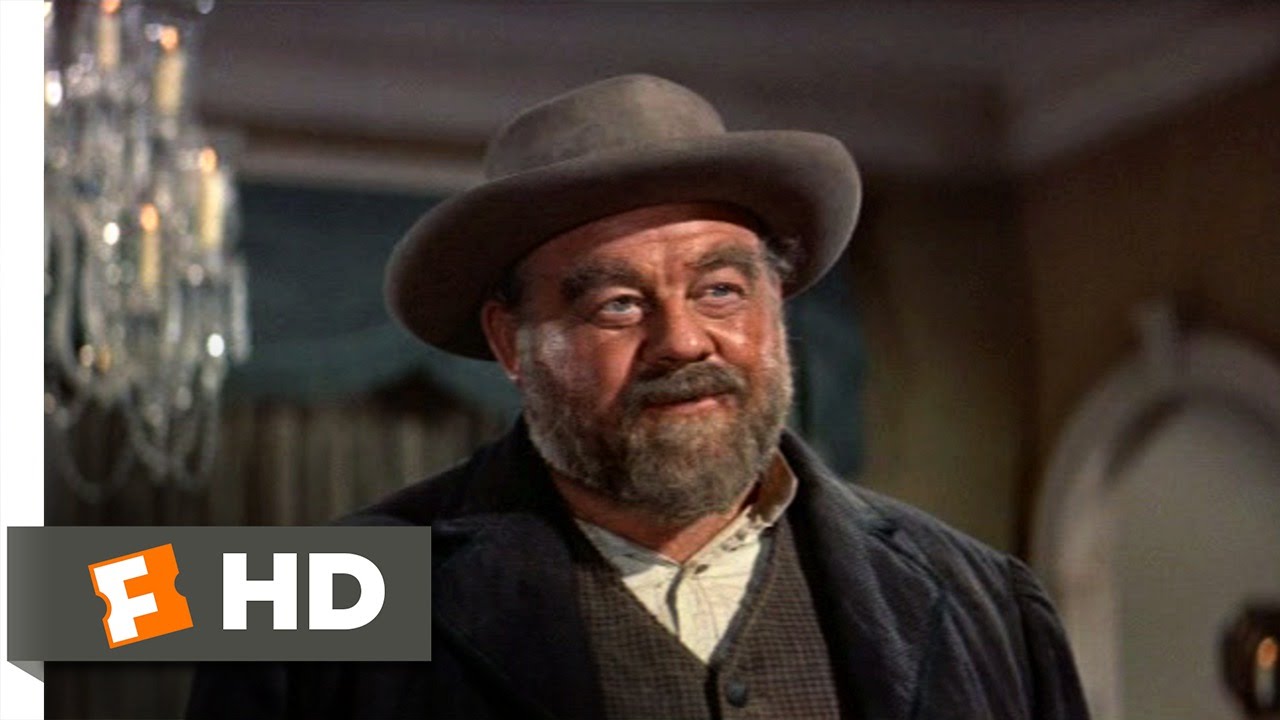This detailed photograph appears to be a still from a TV show or movie set in an old Western style setting, featuring a portly gentleman likely in his late 50s or early 60s. The man, who has a weathered complexion with a ruddy tan and visible wrinkles, is adorned with a salt-and-pepper beard and a matching mustache. He wears a dusty, old-style hat that resembles a cowboy hat but is not quite as tall, and he is dressed in a charcoal gray overcoat layered over a brown plaid vest and an ivory-colored shirt, open at the collar. His attire, combining a darker blue jacket and vest with a lighter shirt underneath, complements his rugged look. The man's full round face and his expression, which carries a slight smile, suggest he is engaged in conversation, his eyes directed off to the right as if listening intently to someone just out of the frame. The background, slightly blurred, indicates an indoor setting with a luxurious, multi-level crystal chandelier hanging from above, draperies with a teal blue valance, and deep tan walls. An entryway door with wood banding and a white ceiling complete the elegant room. In the lower left corner of the photograph, there is a notable Fandango F logo in white on an orange ticket, accompanied by the letters "HD" in large white font. The overall color palette includes shades of charcoal, taupe, and white, adding to the vintage ambiance of the scene.